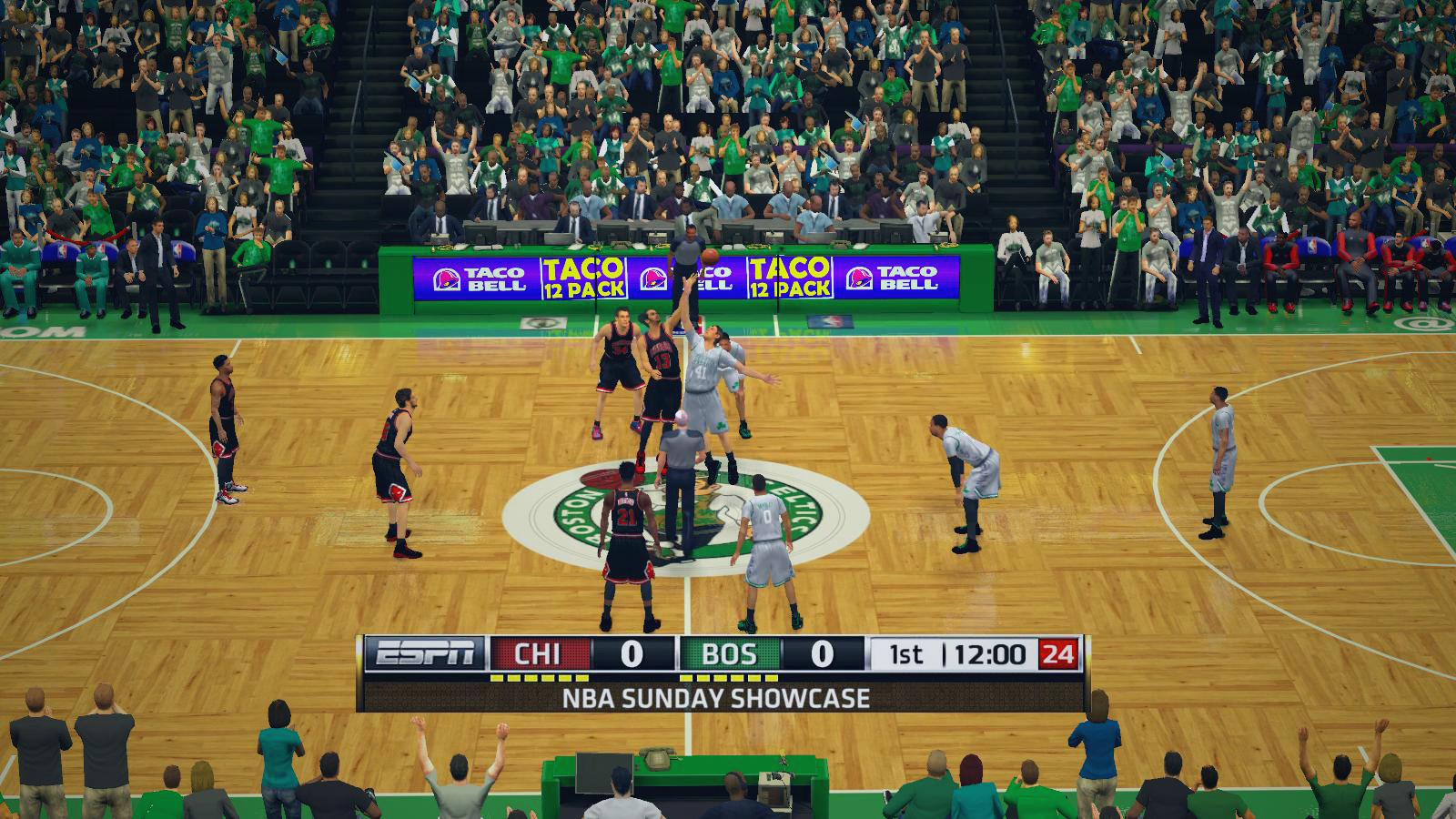The image resembles a scene from a video game, likely a basketball simulation. In the bottom-left corner, the ESPN logo is visible, followed by "Chicago" in white text against a black background displaying a score of zero. Below this, the caption "NBA Sunday Showcase" is present. Near the top of the screen, a green square with white text shows the abbreviation "VOS," indicating zero points in the first quarter. Adjacent to this is a vertical line and the time "12:00," next to a black square with the number "24" in white text over a red background, possibly an advertisement for Taco Bell's Taco 12 Pack.

The court has a wooden floor with white boundary lines, including a large white circle at the center court marked by a central line. The stands are filled with digital spectators wearing predominantly green and white shirts, with some individuals sitting on the bench and others animatedly jumping up and down. Digital athletes, dressed in black or white uniforms, are captured mid-action, leaping into the air to grab the basketball tossed up for a jump ball at the start of the game.